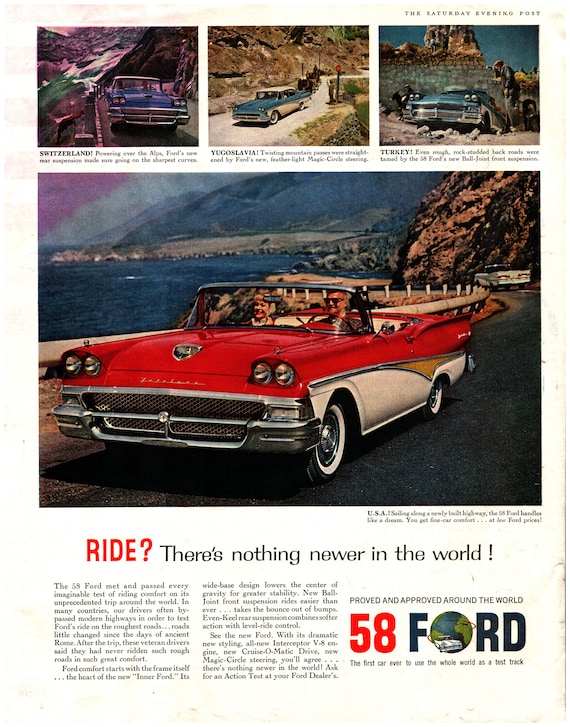The advertisement showcases a classic '58 Ford and appears to be from the Saturday Evening Post. Dominating the center of the page, a striking red and white convertible with a touch of yellow on the side panel is depicted, driven by a smiling couple along a coastal highway, with the ocean and mountains as a scenic backdrop. Above, a panel of three smaller images, aligned horizontally, highlights the Ford in various international locales such as Switzerland, Yugoslavia, and Turkey, showcasing the same model in different settings and colors, predominantly blue with a white top. The top-right corner prominently features the Saturday Evening Post branding, while the lower section of the ad includes descriptive text. It reads in bold red letters, "Ride?" followed by the phrase in black, "There's nothing newer in the world!" Further down, the tagline "Proved and approved around the world" is visible alongside the declaration, "58 Ford, the first car ever to use the whole world as a test track." This composition underlines the Ford's global appeal and durability.